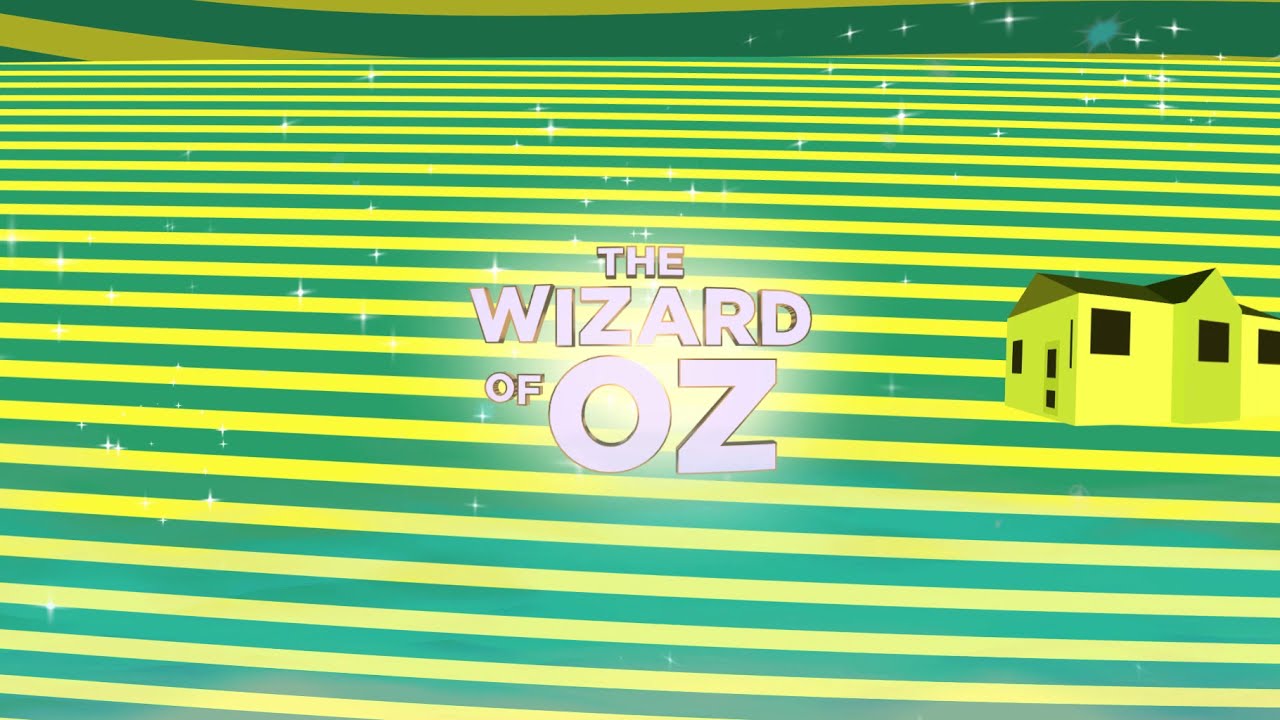This digital poster image for "The Wizard of Oz" features a horizontal rectangular layout with a vibrant background of alternating horizontal yellow and dark green stripes. Dominating the center of the image, the title "The Wizard of Oz" is prominently displayed in capital white letters with a subtle 3D effect and a faint backlight, arranged across three lines with "OZ" in larger font. To the right of this central text, there's a cartoonish depiction of a single-story yellow house with a dark green roof and black windows. Scattered across the image are small, white, twinkling stars, adding a magical touch. Notably, thicker green stripes adorned with white star-like crosses appear along the top, adding depth to the design.